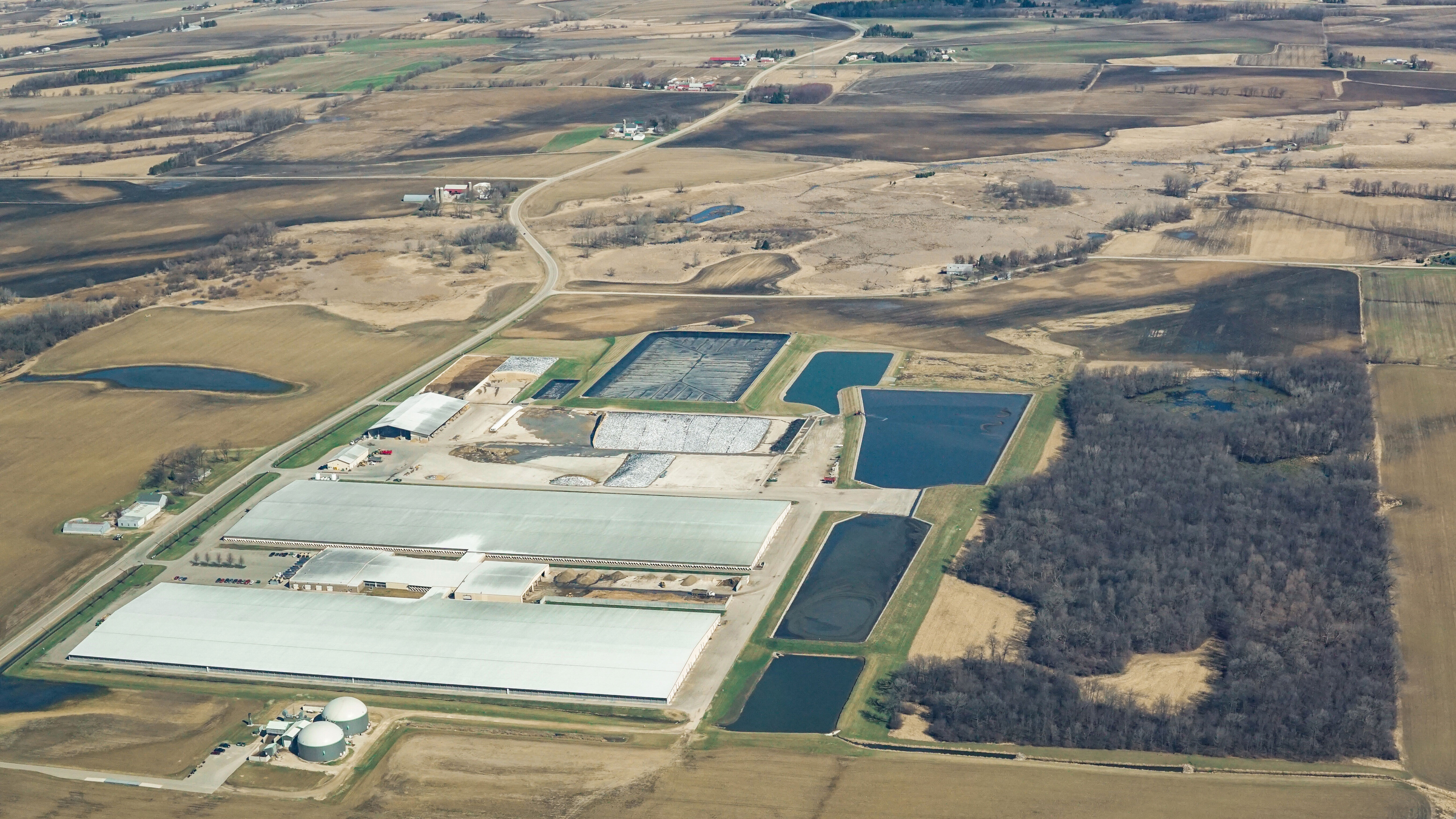This horizontal aerial photograph, likely captured from a plane or helicopter, showcases a wintery landscape composed predominantly of dirt fields arranged in squares and rectangles. The image has a soft, pastel-like glow, potentially enhanced with photo editing software to smooth lines and brighten the scene. The color palette transitions from earthy browns and yellows to hints of dark brown or grayish brush and sporadic areas of blue and silver.

Interspersed throughout the dirt fields are long, gray buildings and a few circular structures that appear to be silos. Some sections feature blue, rectangular formations that might be black tarps. Dirt roads meander through the landscape, adding a sense of structure and connectivity to the otherwise flat and expansive view. The overall effect is a serene yet intriguing tableau of rural terrain, enhanced by thoughtful post-processing that accentuates its inherent beauty and detail.